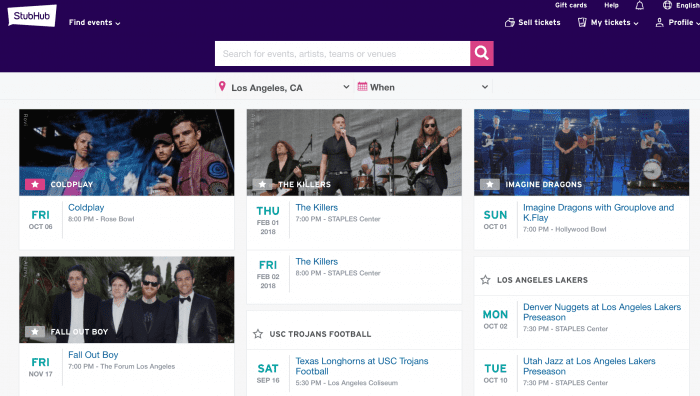In the upper section of the image, there is a large, dark blue box featuring a small white box with the StubHub logo. The box includes the text "Find Events" accompanied by a small downward arrow. Adjacent to this is a search box with a pink end featuring a magnifying glass icon. Additional text in this section reads "Sell Tickets," "My Tickets," and "Profile."

The background is a light blue color, highlighting a small pink pin icon with the text "Los Angeles, California" next to a downward arrow. To the right, there's also a pink calendar icon labeled "When," with another downward arrow beside it.

Below this navigation section, the image showcases several event listings with pictures. The first listing is for Coldplay, highlighted by a pink box with a white star:
- **Friday, October 6th**: Coldplay at 8:00 PM at the Rose Bowl.

The next listing is for Fall Out Boy:
- **Friday, November 17th**: Fall Out Boy at 7:00 PM at The Forum in Los Angeles.

In the middle section, there's a listing for The Killers with two events:
- **Thursday, February 1st, 2018**: The Killers at 7:00 PM at Staples Center.
- **Friday, February 2nd**: The Killers at 8:30 PM at Staples Center.

Continuing downward, another listing features USC Trojans Football:
- **Saturday, September 19th (Tentative)**: Texas Longhorns vs. USC Trojans Football at 8:30 PM in Los Angeles.

The next event highlighted is for Imagine Dragons, with supporting acts Group Love and Kay Flay:
- **Sunday, October 1st**: Imagine Dragons at 7:00 PM at the Hollywood Bowl.

Lastly, there are event listings for Los Angeles Lakers preseason games:
- **Monday, October 2nd**: Denver Nuggets vs. Los Angeles Lakers.
- **Tuesday, October 10th**: Utah Jazz vs. Los Angeles Lakers.